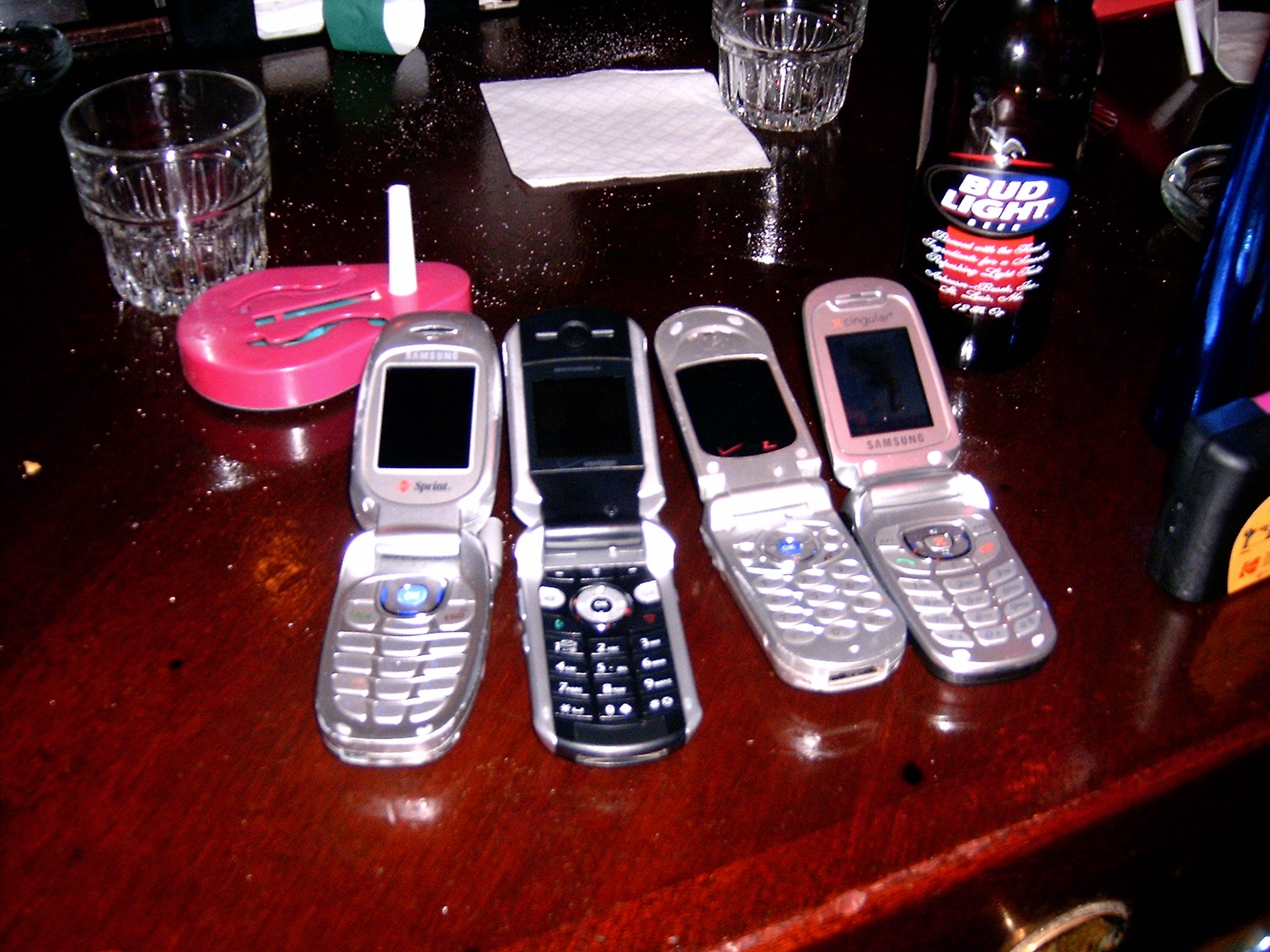The image showcases a lacquered, dark reddish wooden table or desk, possibly located in a restaurant or diner, characterized by its shiny and polished surface with some signs of wear and tear. On the table are four old-school flip phones, all open with tiny screens. One phone displays the Sprint logo, another shows the Samsung brand, while the other two remain unidentified. The flip phones vary in color: two are entirely silver, one is silver with a black trim, and one is silver and pink. Surrounding the phones are an assortment of items, including a folded napkin, two cocktail glasses, and an ashtray just visible at the right edge. There's also a 12-ounce bottle of Bud Light, partially visible without its neck, and a small black container with a yellow label. Additional items include what might be a disposable camera, a pink noisemaker toy with a white handle or antenna, and scattered granules that could be salt or sugar. The overall setting suggests a casual, everyday dining location like a TGI Fridays or a similar establishment.